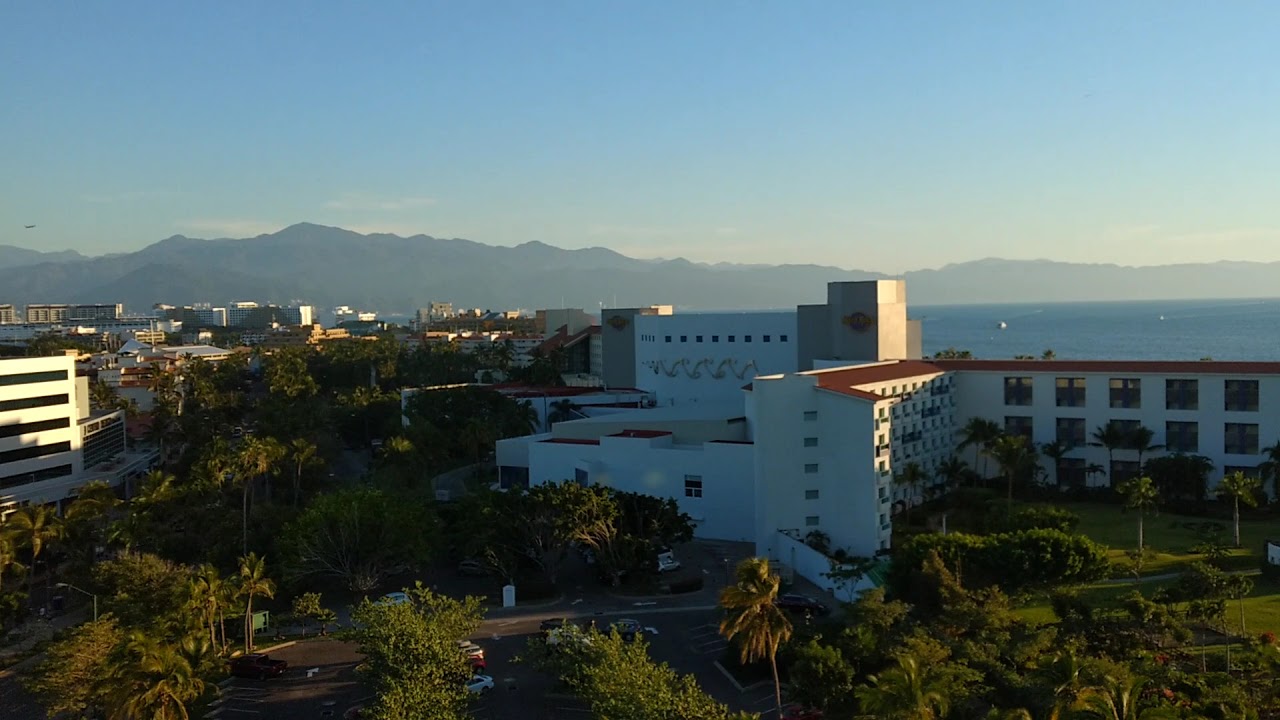The image depicts a cityscape near a coastline or ocean, identifiable by the visible water in the background. Central to the image is a prominent four or five-story white concrete building, likely a hotel or convention center, featuring both large dark windows and numerous smaller ones. Surrounding this main structure are scattered three and four-story buildings. The setting is tropical or at least experiencing pleasant weather, as evidenced by the abundant palm trees, shrubbery, and other lush greenery. 

In the foreground, there is a parking lot filled with cars. Signs and power lines are also visible, adding to the urban scene. The backdrop of the image reveals a range of large hills or mountains, colored in a grayish-blue hue, which contribute to the picturesque landscape. The sky above is a bright blue, slightly hazy, indicating midday with clear and sunny conditions. Additionally, a plane can be seen flying far in the background, enhancing the sense of depth and activity in this vibrant coastal city.